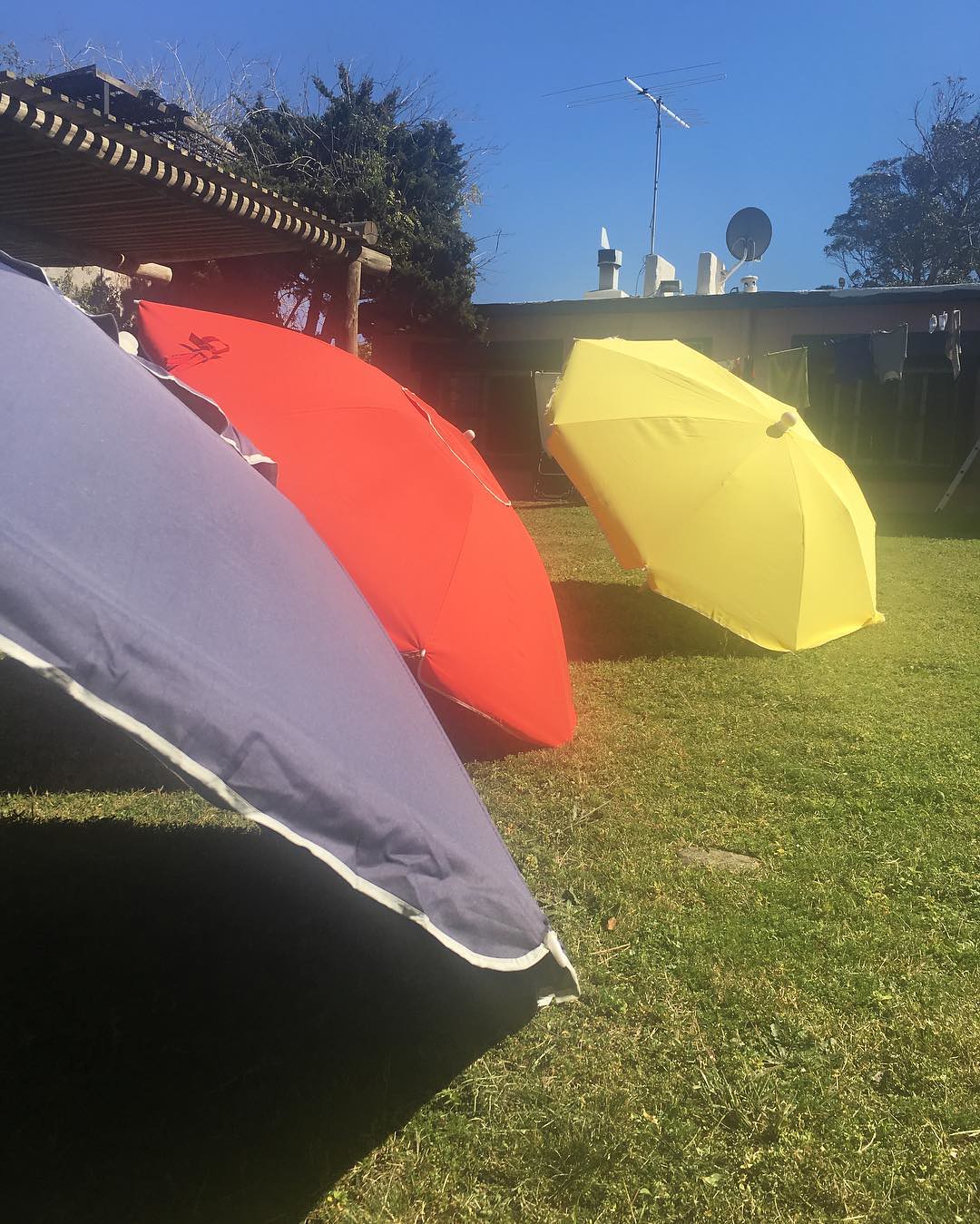The image is a color photograph in portrait orientation capturing a backyard scene. In the foreground, several large, fully-open beach-style umbrellas are resting on the grass. The closest umbrella to the viewer is on the left side of the frame, featuring a purplish-blue hue. Next to it is a vibrant, almost reflective orange umbrella, and further to the right is a yellow umbrella. These umbrellas, used for patio or beach shade, create an arc-like formation across the grassy yard. Behind the yellow umbrella, there's a partially visible structure, possibly a single-level ranch house. This house has a satellite dish, a TV antenna, a metal chimney, and vent pipes on its roof. There is a clothesline stretched across the yard with various items of clothing hanging from it. Additionally, on the left side of the image, partially obscured by the umbrellas, is a wooden gazebo with visible horizontal struts and a vertical pole, likely covering a patio area. The grass in the yard varies in color from darker green patches to lighter, lime green areas further back.